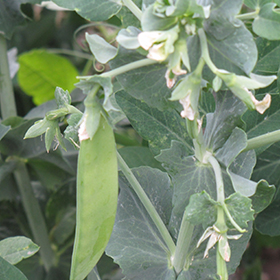The color photograph is a square, outdoor nature shot taken during the daytime, likely on a cloudy day, from an above and slightly angled perspective. The image captures a small plant with varying shades of dark green leaves, indicating the presence of more than one type of foliage. The leaves are small and some appear to have been chewed by insects. Among the leaves, there are branches with small, white flowers in different stages of blooming; some are opening while others remain as buds. Particularly noticeable is a bright, yellowish-green leaf in the upper left corner, which stands out against the darker, shadowed background. Additionally, there is a pea pod on the left side of the plant, lighter green in color and pointing downward. In the background, other small plants with similarly colored leaves can be seen, although they are mostly obscured by shadows, with some grass pieces visible as well.